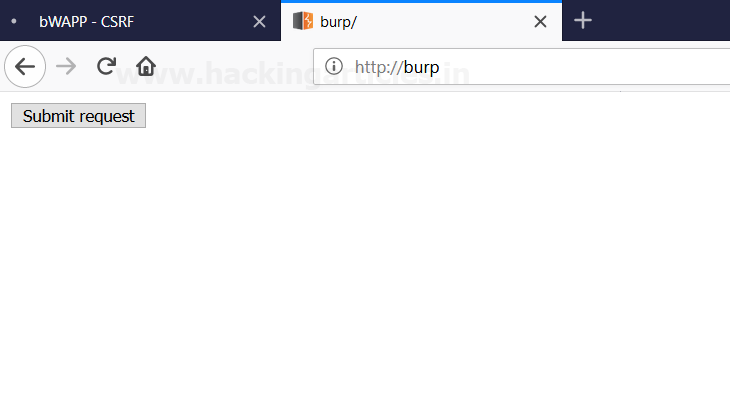The image depicts the top section of a web browser or a web-based application interface, with a focus on its detailed elements and layout. The interface is noticeably wider than it is tall, approximately five to six times as wide.

Starting from the top, the user interface includes the typical web browser controls – back, forward, reload, and home buttons – along with an address bar where the current website URL is displayed. The browser is open to a website named "BURP."

In the tab section of the browser, there are two distinct tabs. The first tab, which is not selected, features a dark blue background with white text that reads "bWAPP-CSRF." This text is mostly uppercase with the exception of the 'b' which is in lowercase. To the right of this text is a small 'X' icon used to close the tab.

The second tab, which is the active tab, has a white background and black text stating "BURP." To the right of this text is a backslash symbol, and to the far right is another 'X' icon, used for closing the active tab. Additionally, there is a 3D cube logo featuring gray and orange faces located to the left of the text.

The bottom section of the image coincides with the browser's navigational icons and the website address bar suggesting that the browser is currently displaying the BURP web page.

Overall, the image shows a clean and detailed view of a web browser interface with a blue accented tab layout and a prominent active website tab indicating the current page as "BURP".